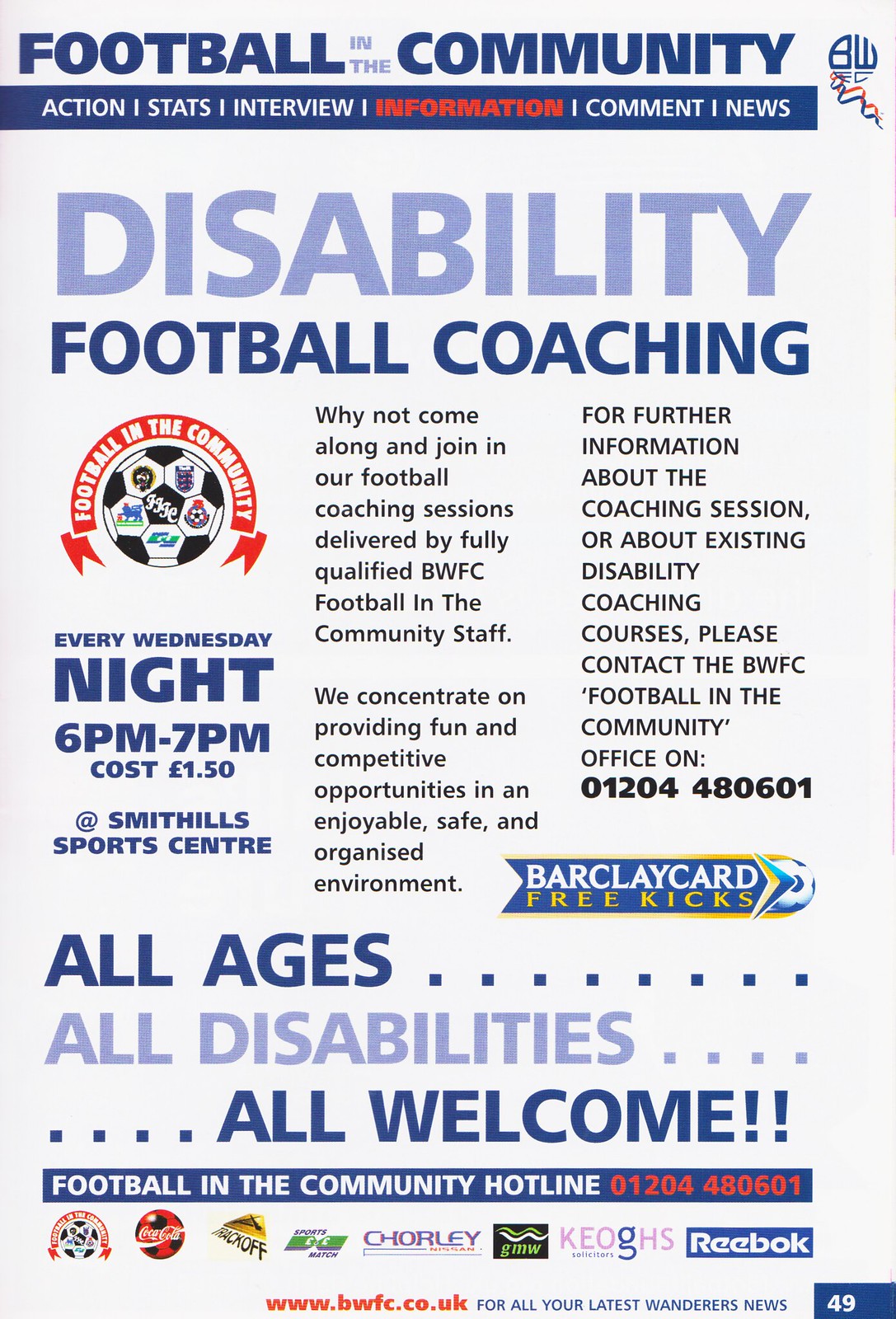The image is a white background poster promoting a community-focused event in the United Kingdom, titled "Football in the Community," prominently displayed in blue capital letters at the top. Below this, a blue banner highlights segments such as "Action," "Stats," "Interview" in white text, and "Information" in red, followed by "Comment" and "News" in white. A light blue section emphasizes "Disability Football Coaching," encouraging people to join weekly football sessions conducted by fully qualified BWFC community staff. The sessions promise a fun, competitive, and safe environment and are open to all ages and disabilities, taking place every Wednesday from 6 PM to 7 PM at Smith Hills Sports Centre, costing £1.50.

On the left, there is an image of a football encircled in red with the text "Football in the Community." The poster details how to contact the BWFC football in the community office for more information about the coaching. It provides the hotline number 01204 480601 and references the website www.bwfc.co.uk. A small blue banner at the bottom reiterates the hotline details.

Sponsorship logos displayed include Coca-Cola, Reebok, Barclaycard Free Kicks, Track Off, Sports Match, Chorley Nissan, GMW, and Keogh's Solicitors, all listed near the bottom. Additionally, for the latest news on Wanderers, visitors are directed to read further information on the provided website.

The poster vividly combines information and visual elements to foster community engagement through accessible and inclusive football coaching sessions.